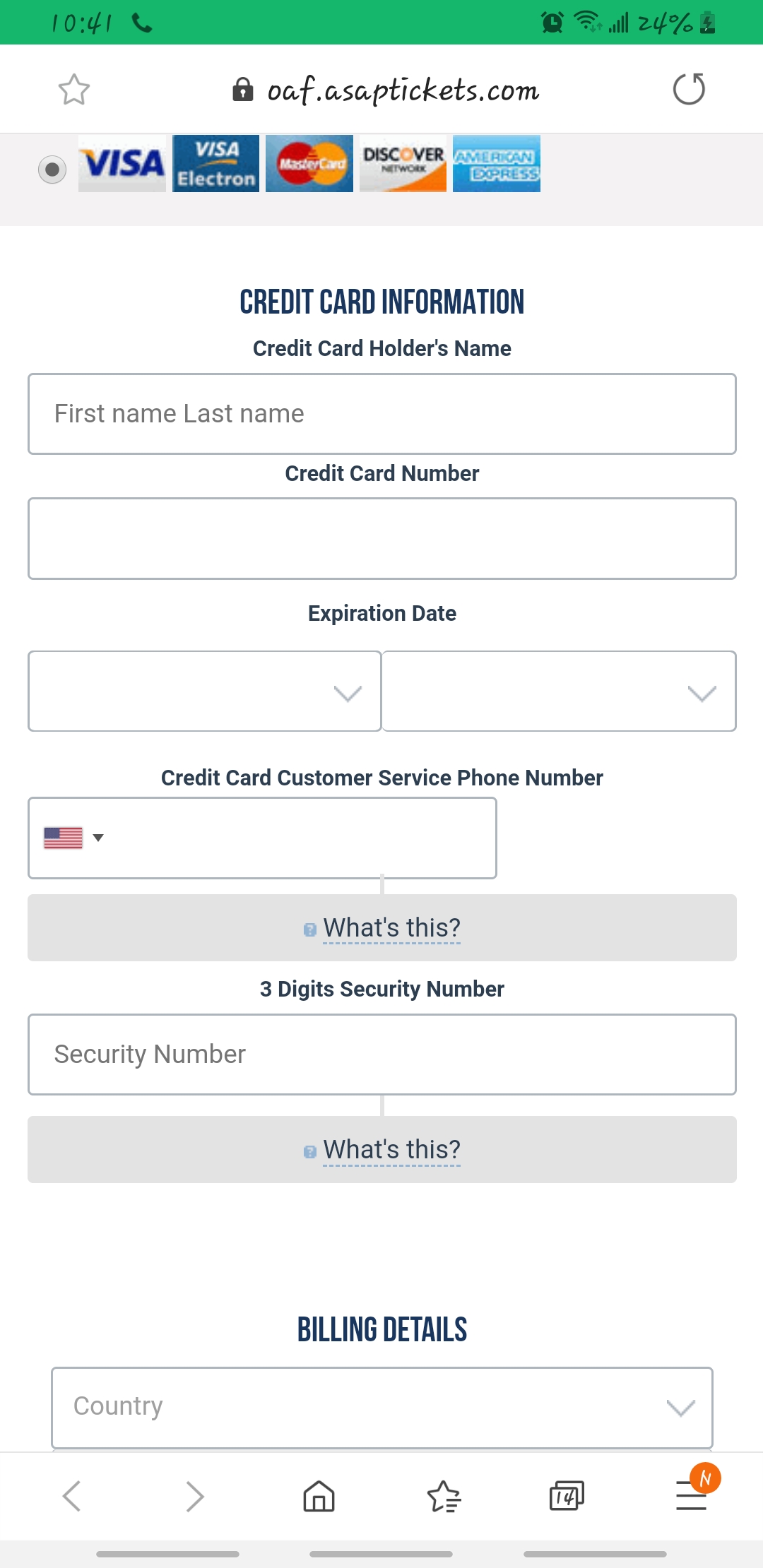In this detailed screenshot of a cell phone displaying a payment application, the time at the top reads 10:41. To the right of the time, a telephone icon is followed by a series of icons indicating various functionalities, and the battery life is at 24%, depicted in green. These elements are enclosed in a green rectangular box.

Centered below this green box is a secure website URL, designated by a lock icon in black next to "oaf.asaptickets.com." Adjacent to the URL, on the right side, is a reload button, while on the left is a favorite button marked with a star icon.

The main section of the screenshot is devoted to payment methods, specifically credit card options. The available options include Visa, Visa Electron, MasterCard, Discover Network, and American Express, each accompanied by their respective logos. A dot inside a circle next to the Visa logo indicates that Visa has been selected as the payment method. This entire section is encompassed in a gray rectangle labeled "Credit Cards."

Following this, the interface prompts for credit card information. The requested details include the cardholder’s name, with corresponding input fields for the first and last name, all displayed in black capital letters. Next, it asks for the credit card number, followed by an input box to enter the information. 

Further down, there are boxes to input the card's expiration date, split into two fields for the month and year. Additionally, the interface provides a customer service phone number for credit card assistance. Right at the bottom, a box containing the United States flag is displayed, likely indicating the country code or locale setting for the customer service.